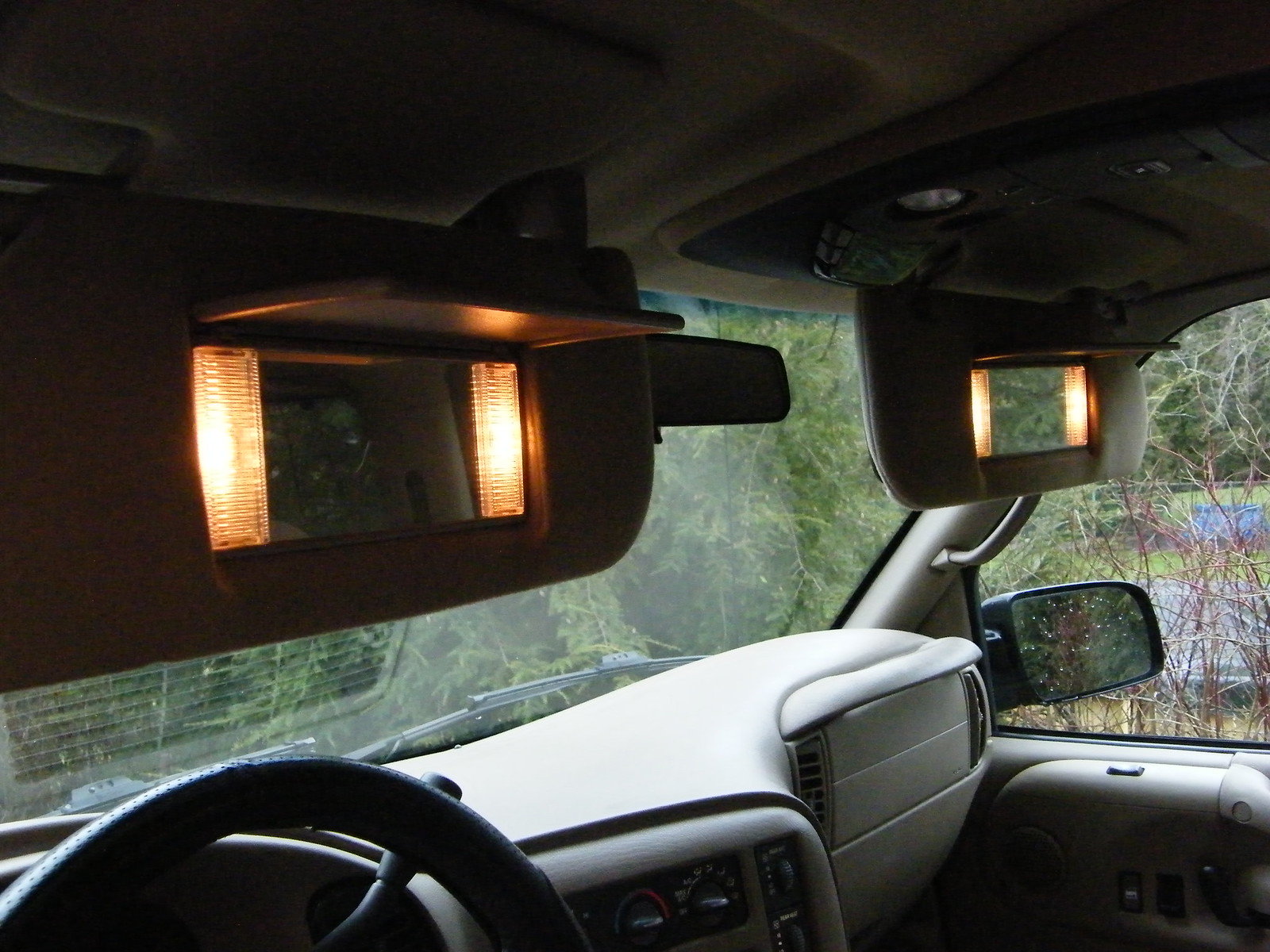This color photograph captures the interior of a car during daylight, showcasing a detailed and layered composition. The primary focus lies on the down visors on both the driver's and passenger's sides, each featuring a vanity mirror lit by four orangish-yellow lights, casting a soft glow. The image is taken from an angled view on the driver's side, looking right over the passenger side dash, emphasizing the vehicle's gray and tan interior, which is relatively clean. Visible are the top section of the steering wheel in the bottom left corner, part of a tan vinyl console, and a shifter next to the steering wheel.

The scene outside the car includes a view through the lower part of the front windshield and the passenger side window, revealing a yard filled with tangled trees, shrubbery, and potential shapes of tarps. Reflections of greenery are noticeable in the passenger side mirror. The photograph also includes elements such as the rearview mirror's edge, windshield wipers, and the grates for the air vents reflecting on the windshield glass. The contrast between the darkly lit car interior and the bright exterior creates a visually interesting interplay of light and shadow in the image.